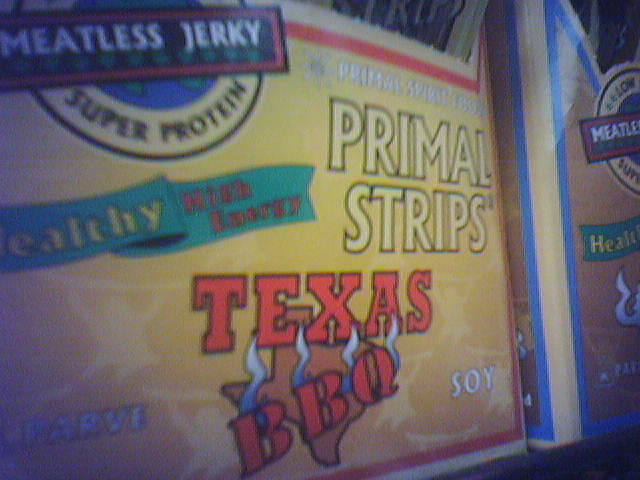The image features packaging for Primal Strips, a type of meatless jerky. The bottom portion of the package displays a yellow square with the descriptor "Soy" prominently. In the bottom left, there is some additional text, though it's unclear. The top left corner of the packaging reads "Meatless Jerky," and beneath this, "Super Protein" is highlighted.

A blue ribbon on the package signifies that the product is "Healthy." To the right, the brand name "Primal Strips" is visible. Further to the left, the flavor "Texas BBQ" is clearly indicated, accompanied by an orange Texas T symbol with white wavy lines.

The background features outlines of multiple people holding spears, which add a primal aesthetic to the design. The top left section of the packaging has a red border with stripes, while the right side includes a blue outline, providing a bold and contrasting visual appeal.